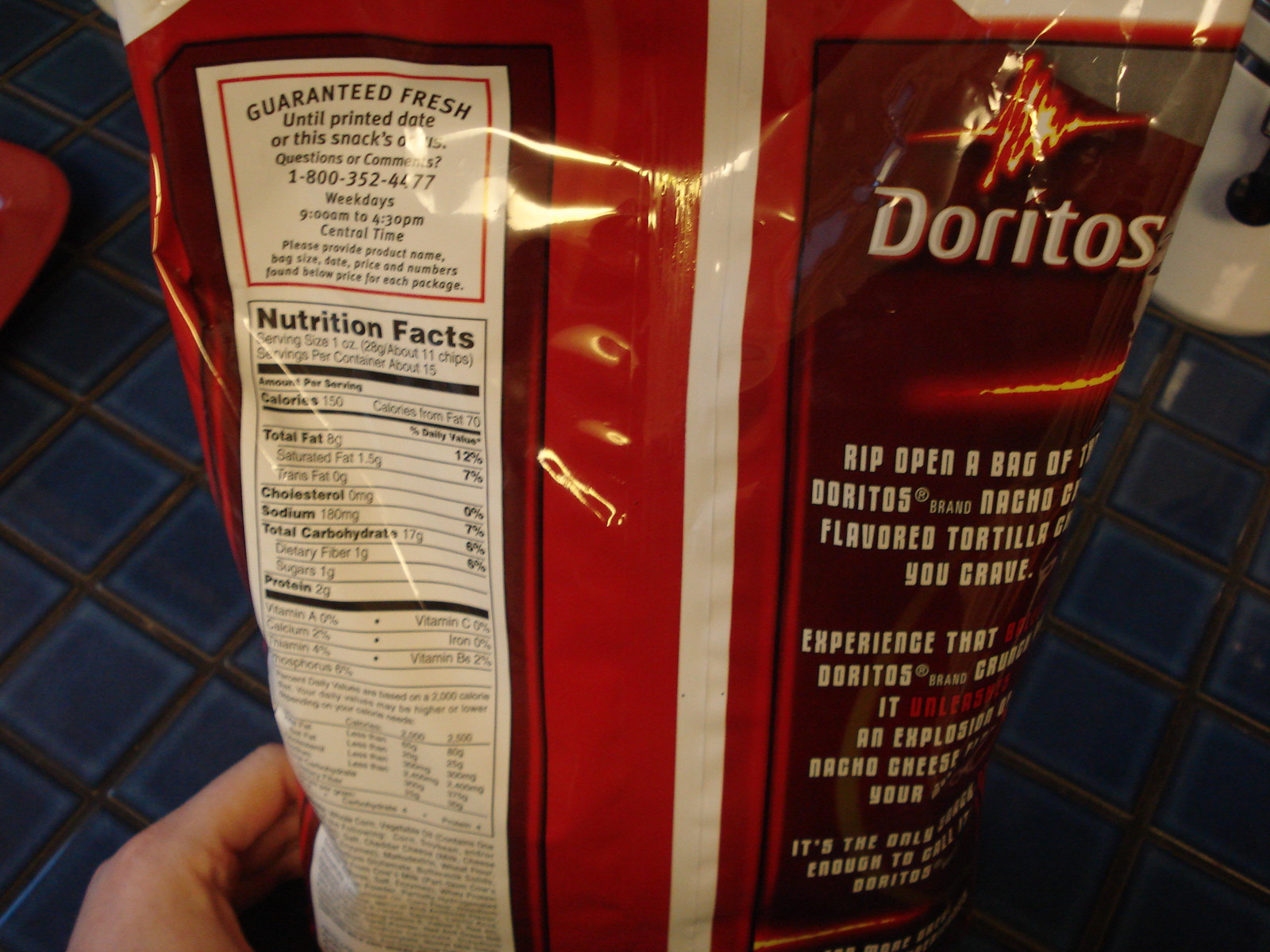In this rectangular photograph, we see a close-up view of the back of a bag of Doritos. A Caucasian hand is positioned in the lower left corner of the image, gripping the lower part of the bag. The hand is visible from the side, with the pointer finger wrapped around the bag and a part of the palm exposed.

The top right corner of the Doritos bag displays the brand name "Doritos," accompanied by an image that appears to be a flame. In the top left corner, there is a white label that reads, "Guaranteed Fresh Until Printed Date or This Snacks. Questions or comments," followed by a helpline number, "1-800-352-4477," with availability listed as weekdays from 9 AM to 4:30 PM. Below this label, the nutritional facts are printed, indicating a serving size of 1 oz. and approximately 15 servings per container.

The primary color of the bag is red, except for the white nutritional information, printed text, and a white vertical stripe running down the center on the back. The bag is held over a background that features black square tiles, likely indicating a countertop.